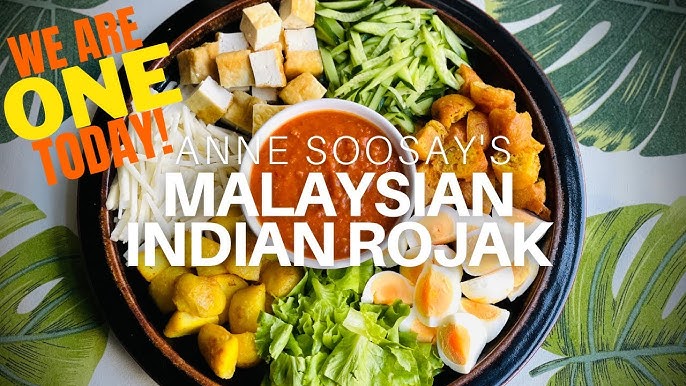The image presents a vibrant and enticing bowl of "Ann Suse's Malaysian Indian Rojak," highlighted by overlaid text. The bold, colorful fonts read "We Are One Today!" with "We Are" in orange, "One" in yellow, and "Ann Suse's Malaysian Indian Rojak" boldly displayed in white. The bowl, set on a placemat featuring vivid monstera leaves in shades of green and white, contains an appealing array of ingredients divided into sections. Starting from the top and moving clockwise, there are fresh cucumber slices, crispy croutons, chopped boiled eggs, shredded lettuce, potentially gnocchi, a golden fried element possibly being tofu, and small green vegetables. At the center of the bowl, there's a rich, red dipping sauce that appears tomato-based, ready for the assorted items to be dipped in. The background's leafy design enhances the fresh, vibrant presentation of this served Malaysian Indian dish.